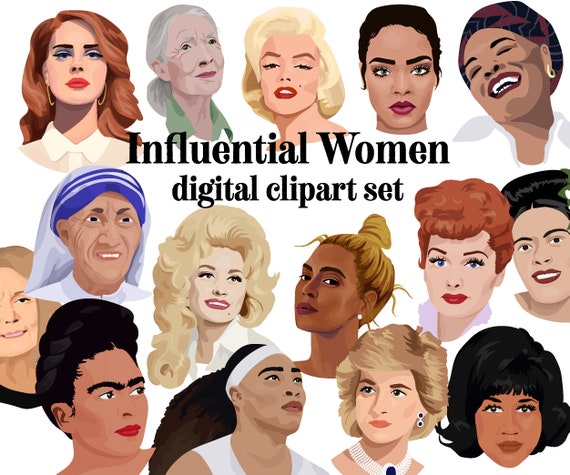The image depicts a digital clip art set titled "Influential Women." At the top, black text reads "Influential Women Digital Clip Art Set." Centrally featured are 15 animated faces of women, arranged in three rows. The top row showcases five faces, the middle row contains six, and the bottom row displays four. The characters vary in age, skin tone, and hair color, reflecting a diverse representation. The background is white, providing a clean and unobtrusive backdrop that accentuates the vibrant and varied details of each animated face.